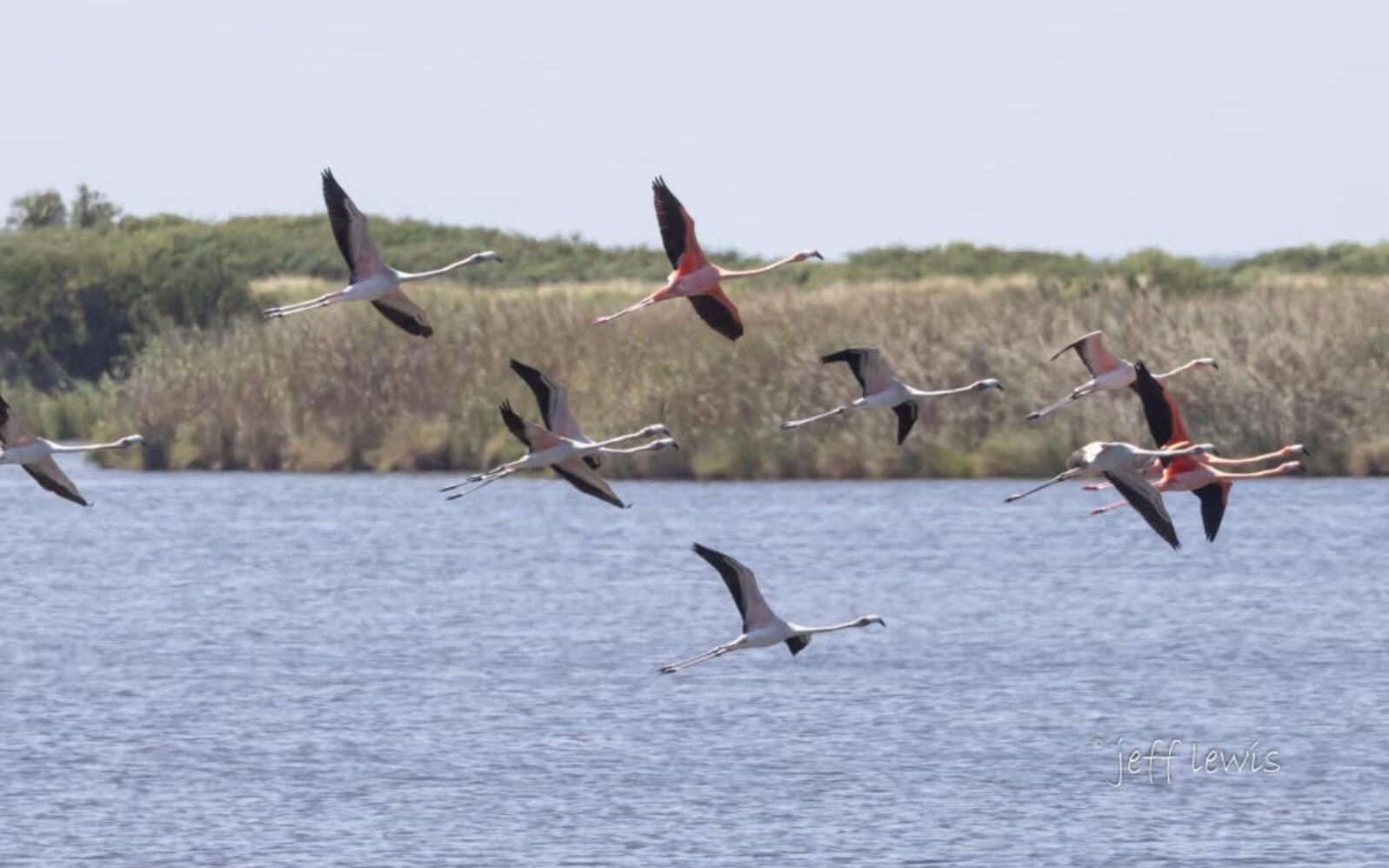In the image, a flock of eleven birds is captured mid-flight over a body of water, likely a lake or river. The birds exhibit the distinctive features of flamingos, with long necks, elongated legs, and beaks characteristic of the species. Their plumage varies between shades of pink, white, and gray, adorned with black highlights on the tips and undersides of their wings. The water beneath them displays a range from lighter to darker blue hues, suggesting light currents.

In the background, the landscape features a bank with a blend of green and brown vegetation, marking it as likely summer. The greenery includes grass and small shrubs or trees, although these elements appear blurry and indistinct. The sky above is mostly clear, exhibiting a light blue tone with a hint of haze. The image also contains a watermark in the bottom right corner with the text "Jeff Lewis" written in white.